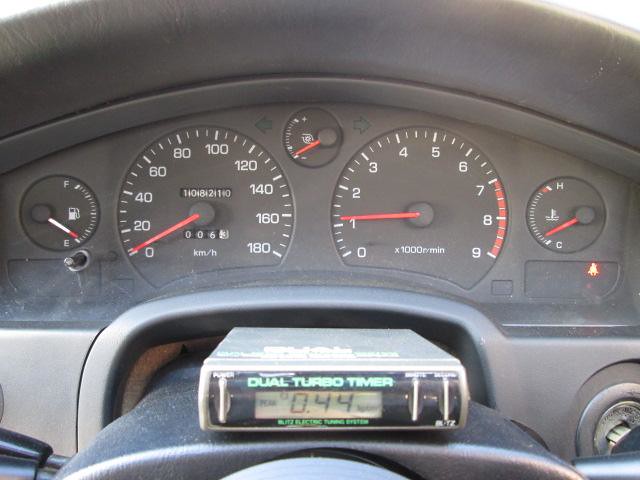The photograph provides a close-up view of the dashboard of an early to mid-1990s automobile, which is currently turned on and idling. The tachometer indicates the engine is idling just above 1,000 RPMs. The gauges on the dashboard show key readings: the gas gauge is near empty, the speedometer is at zero, and an unlabeled gauge with an unfamiliar symbol is centered at the top. Additionally, the oil temperature gauge shows a reading slightly above "C" for cold. A single dashboard light, the seatbelt indicator, is illuminated. In the bottom right corner, part of the car key is visible in the ignition. Prominently displayed in the foreground is a device labeled "Dual Turbo Timer," showing a numeric reading of 0.44 on an old-school LCD screen. Below this, though slightly obscured, the text reads "Electric Tuning System."